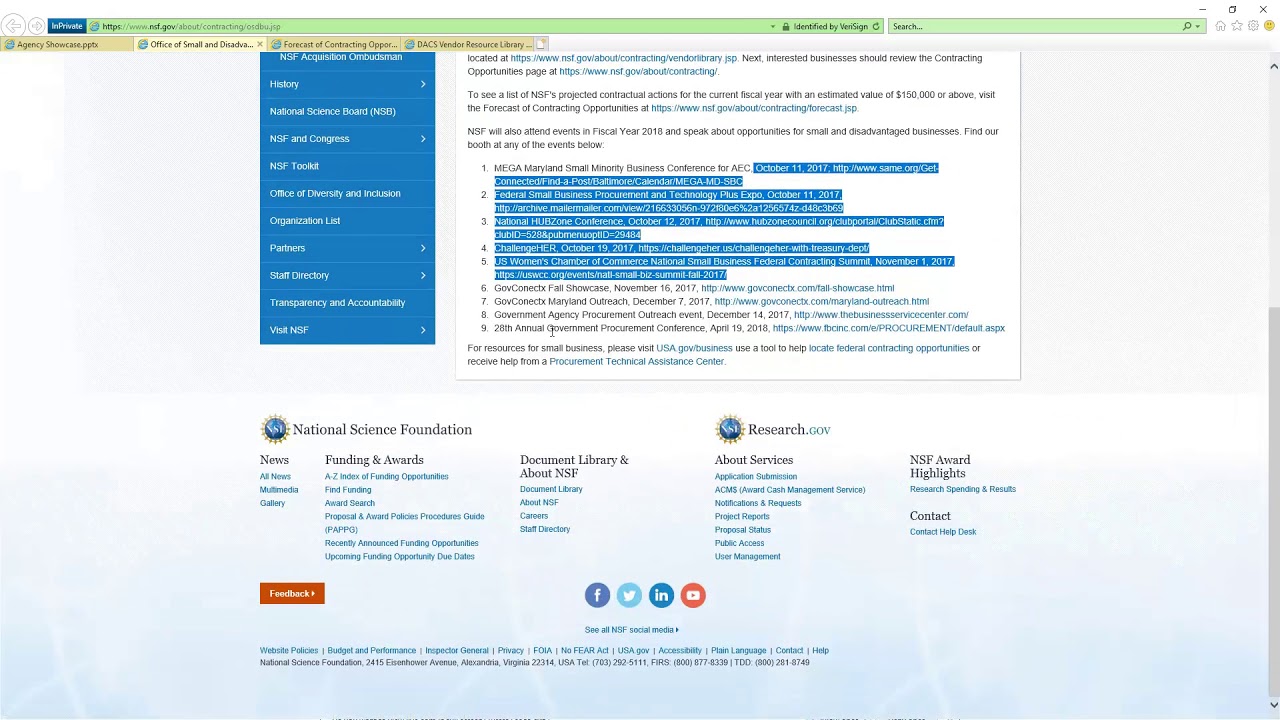At the bottom of the web page, several social media and external links are displayed, including icons for Facebook, Twitter, Indeed, and another unidentified link. Below these icons, there is text indicating this is the website for the National Science Foundation (NSF), accompanied by an emblem and a link to research.gov. Additional links provided are for "Contact," "About," "Services," "NSF Award Highlights," "Document Library," "About NSF," "Funding and Events," and another unclear option.

Moving upwards, the page features a green menu bar at the top, though the text within this bar is too small to be legible. Directly beneath the green bar, there is a yellow tabbed section with four unspecified options. None of these tabs appear to be actively selected. Further down, a blue rectangular box functions as a menu with arrow dropdowns. One of these dropdowns is expanded, revealing a substantial amount of text and numerous highlighted blue links, which are also too small to read clearly.